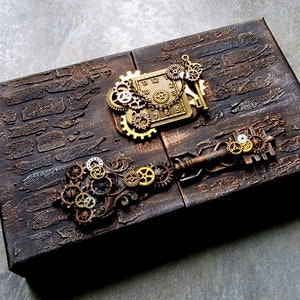The image displays a steampunk-themed wooden chest on a gray surface. The chest is approximately the size of a shoebox with intricately etched brown wood, resembling the texture of bark or brick. The top of the chest is adorned with an array of interlocking gears in gold, bronze, and yellow shades, some of which form a clock-like pattern with numerals from 12 at the top, then 1 through 11 arranged around it. Additionally, there's a section towards the bottom of the lid where gears and sprockets are aligned in a manner evocative of an old-fashioned key. The box is shown tilted diagonally, with parts of its corners cut off in the frame, highlighting its ornate and mechanical decorations.